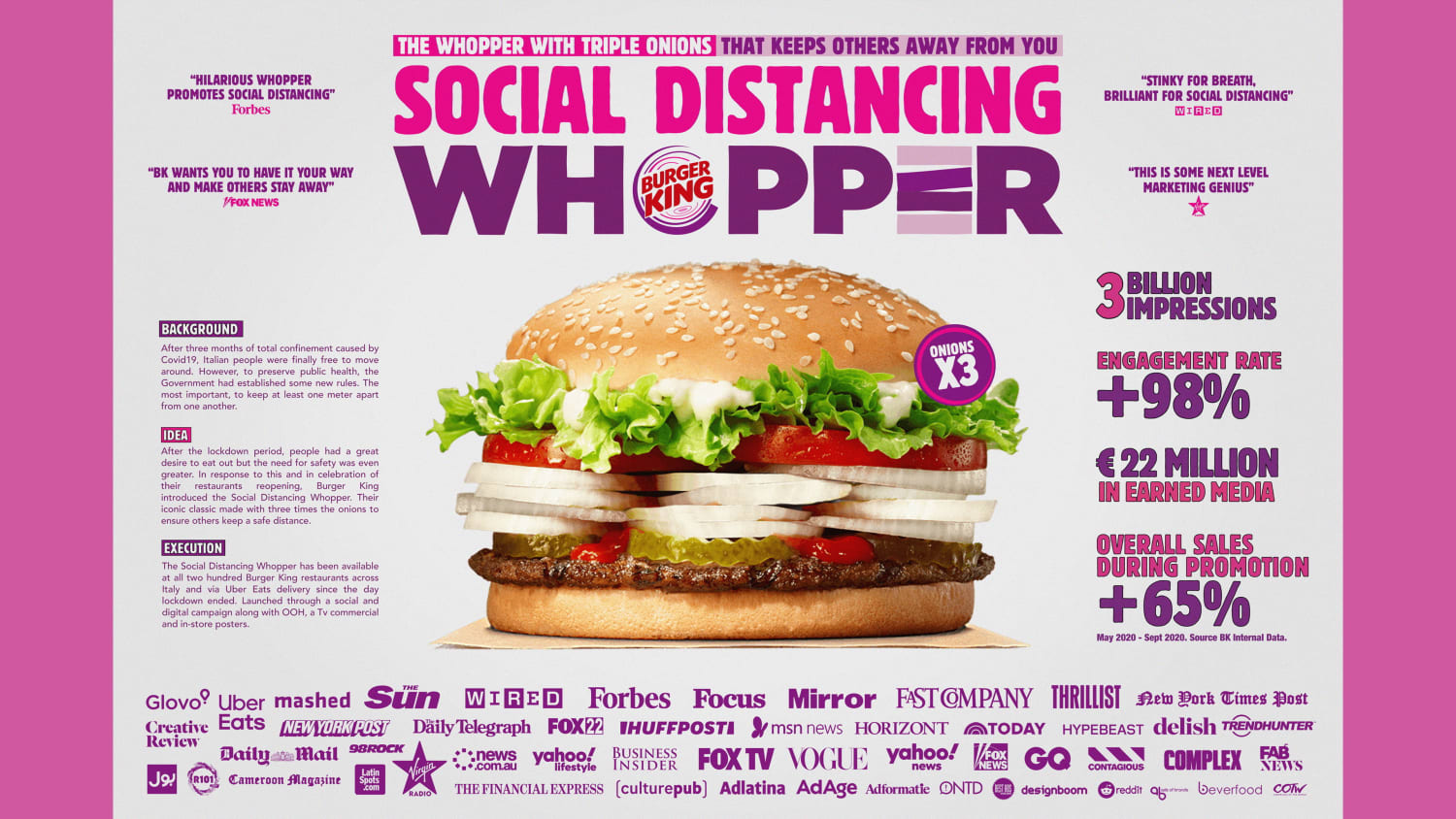The advertisement for Burger King showcases the "Social Distancing Whopper" on a light background bordered by vertical pink or lilac bars. At the top center, within a pink box with white text, it reads "The Whopper with Triple Onions," followed by a light purple box containing the phrase "That keeps others away from you" in dark purple text. Below, in large all-caps pink letters, it says "Social Distancing," and beneath that is the word "Whopper" in purple font, with the 'O' replaced by the Burger King logo and the 'E' styled as two patties between buns. The central image is a vibrant, full-color photo of the Whopper, prominently featuring triple onions among its layers of lettuce, tomatoes, pickles, ketchup, and a sesame seed bun. Flanking this image are columns of text—on the left, detailed paragraphs extolling the Whopper's virtues and humorous aspect, and on the right, impressive statistical data like "three billion impressions." At the bottom, various logos of media outlets highlight extensive coverage of this innovative marketing campaign.